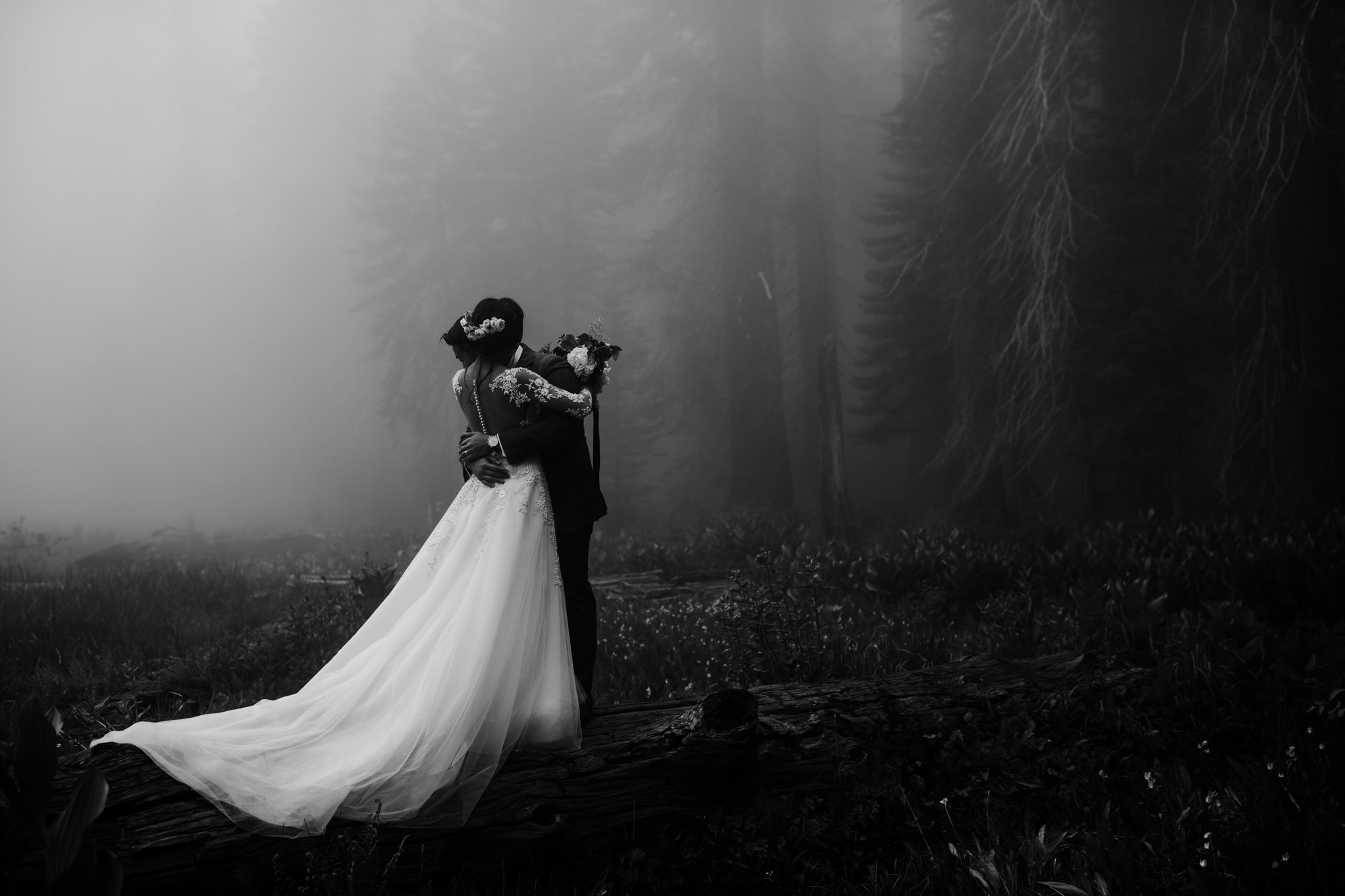In a deeply dramatic black-and-white wedding photograph, a couple stands in a misty outdoor setting, embraced in a tender hug. The bride, positioned on the left, wears a long, white wedding dress adorned with lace on the sleeves, her hair elegantly pulled back into a ponytail, and she grasps a bouquet of flowers. The groom, partially hidden behind her, is clad in a black tuxedo. Their faces are obscured as they share a kiss, adding to the intimacy of the moment.

The background is ethereal and haunting, with tall, dark, and thick pine trees enveloped in a swirling mist, creating a murky, almost eerie ambiance. A small field with short green vegetation, bushes, and wildflowers surrounds the couple. A fallen tree trunk lies beside them, enhancing the rustic feel of the forest floor. On the right side, the photograph is almost entirely dark, contrasting with the foggy left side where the forest appears even more mysterious and enigmatic. The overall underexposed quality and the mist lend an almost somber and atmospheric tone to the wedding photograph, making it uniquely haunting and memorably striking.